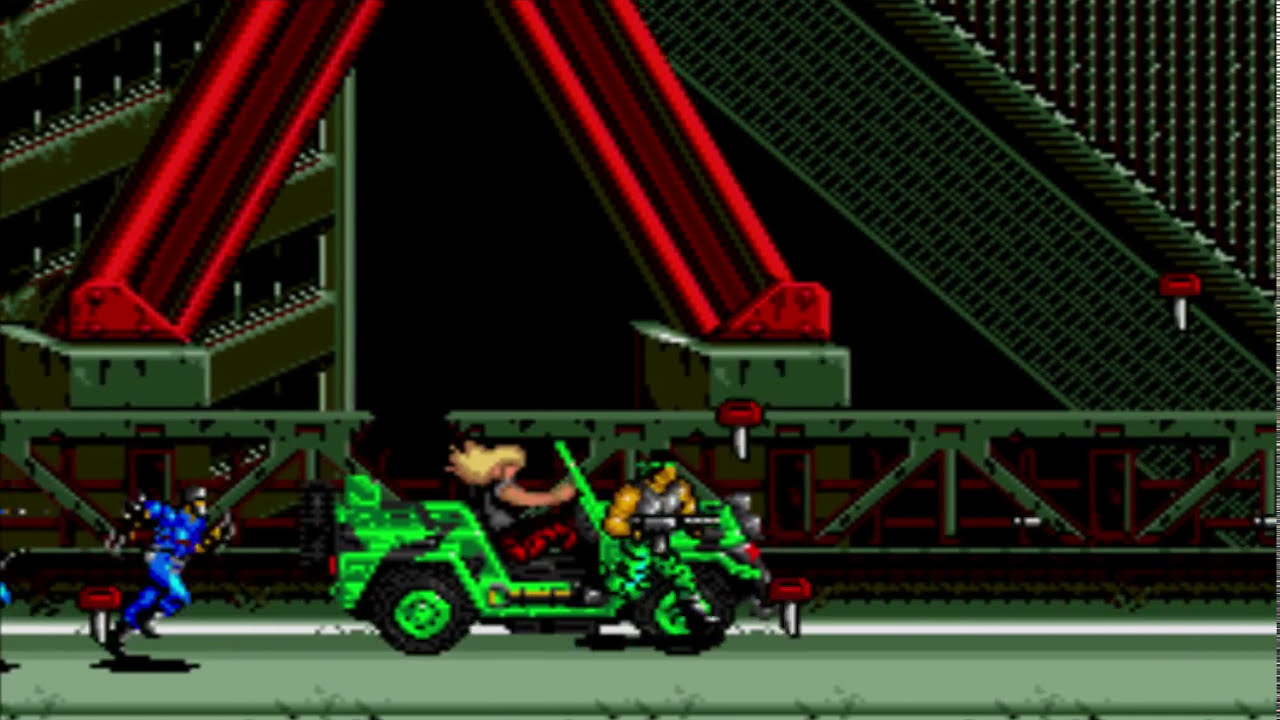The image is a detailed screenshot from the retro-style 16-bit video game, Midnight Resistance for the SEGA Genesis. The scene features a pixelated and somewhat undetailed art style with a limited color palette. At the forefront, there's an open-top, green jeep with black stripes and rims. Driving the jeep is a woman with long blonde hair flowing behind her, wearing red pants and a short-sleeved gray vest. Hanging off the side of the jeep is a muscular man with black hair donning a bright neon green headband, green camo pants, and a white tank top, brandishing a gray machine gun. They're on a flat, greenish-gray concrete road, likely part of an industrial area, identifiable by large steel supports—some greenish, others bright red—and a metal railing or fence. In pursuit, a soldier dressed in a blue suit with black gloves and sleeves is running, adding to the intense action of the scene, all set against a stark black background.